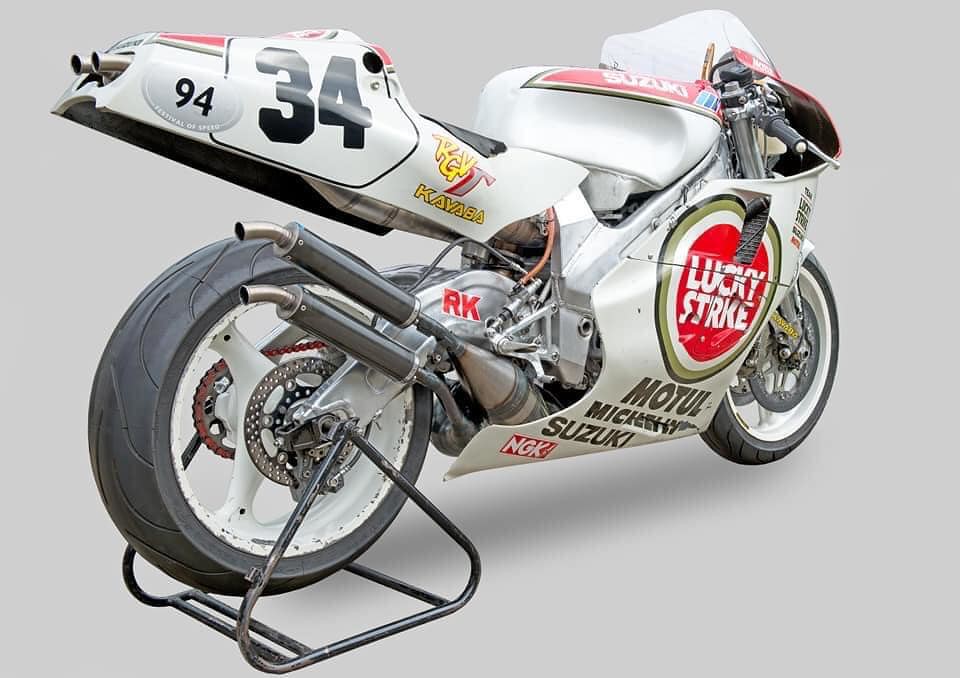The image showcases a sleek, white racing motorcycle positioned on a stand, giving a side view. Prominently featured on the bike are various racing decals and advertisements. At the back, a large number "34" is displayed, accompanied by a smaller "91". The front section, below the wheel, exhibits a red circle with white letters spelling "Lucky Strike", and beneath it, the text reads "Model Suzuki NGK". Additional branding includes "RK" on a metal part of the motorcycle. The black seat has yellow lettering underneath that reads "RGV Kawaba", with a capital letter "T" embedded in the text. The motorcycle also features two side pipes and visible metal elements within the wheels. The word "Suzuki" is clearly written on the top of the bike, further emphasizing its racing pedigree.